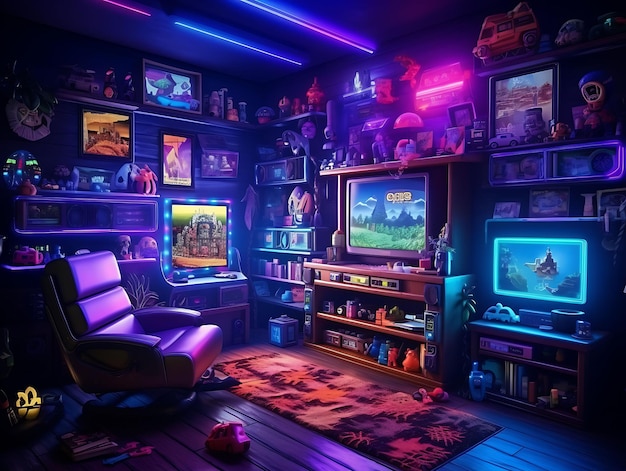This detailed scene captures a cozy, vibrantly decorated gaming or TV room. At its center, there's a comfortable, brown leather chair surrounded by various books. The space is characterized by its dark yet colorful ambiance, illuminated with RGB blue and pink neon lights, which string around framed pictures and cast a vibrant glow across the room. The ceiling also features these neon lights, enhancing the room's playful, energetic vibe.

The wooden floors and walls, the latter lavishly adorned with an array of framed artwork, shelves, and decorations, add warmth to the space. These shelves house an eclectic mix of items, including art pieces, toys such as miniature cars, and other quirky knickknacks. 

Several computer screens add a modern touch, their glowing displays contributing to the room's futuristic aesthetic. An entertainment center stands against one wall, likely holding consoles and a variety of gaming equipment. 

In the middle of it all lies a rectangular rug, woven with shades of orange, black, and tan, lying before a centrally positioned TV. This carefully designed space, with its blend of colorful lights, cozy furnishings, and diverse decorations, provides an inviting atmosphere perfect for gaming, relaxation, and entertainment.